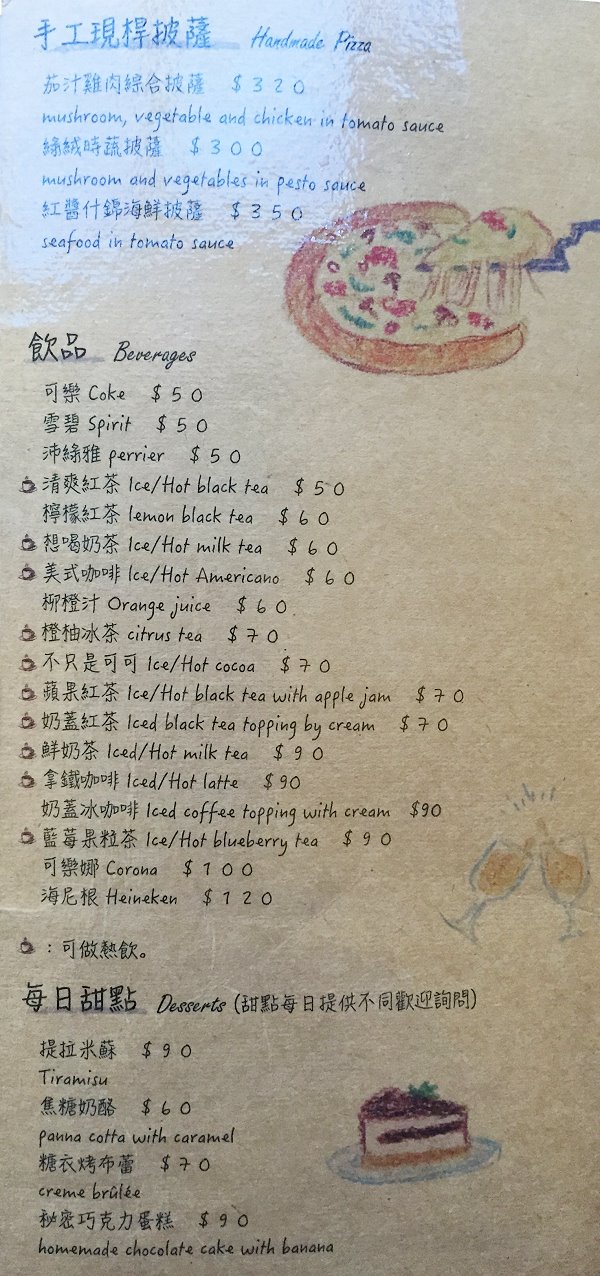The menu, likely from an international restaurant, features an artistic layout with hand-drawn illustrations of various food items set against a beige background with black font. The text is primarily in an Asian language, interspersed with English descriptions. 

At the top of the menu, the highlighted dish is handmade pizza, available with:
- Mushroom, vegetable, and chicken in tomato sauce
- Mushroom and vegetables in pesto sauce
- Seafood in tomato sauce

The beverage section, priced at $50, lists:
- Coke, Sprite, Perrier
- Iced or hot black tea, lemon black tea, iced or hot milk tea
- Iced or hot Americano

For $60, the beverages include:
- Orange juice, citrus tea, iced or hot cocoa
- Iced or hot black tea with apple jam
- Iced black tea topped with cream
- Iced or hot latte
- Iced coffee topped with cream
- Iced or hot blueberry tea

The menu also offers beer options such as Corona and Heineken.

The dessert selection features:
- Tiramisu
- Panna cotta with caramel
- Crème brûlée
- Homemade chocolate cake with banana

The Asian symbols accompanying the text emphasize the menu's international flair. At the bottom, the illustrations include:
- A piece of cake, likely tiramisu or crème brûlée
- Two wine glasses clinking together, symbolizing a celebratory toast
- A pizza slice being lifted by a spatula, showcasing gooey cheese stretching from the slice to the pizza.